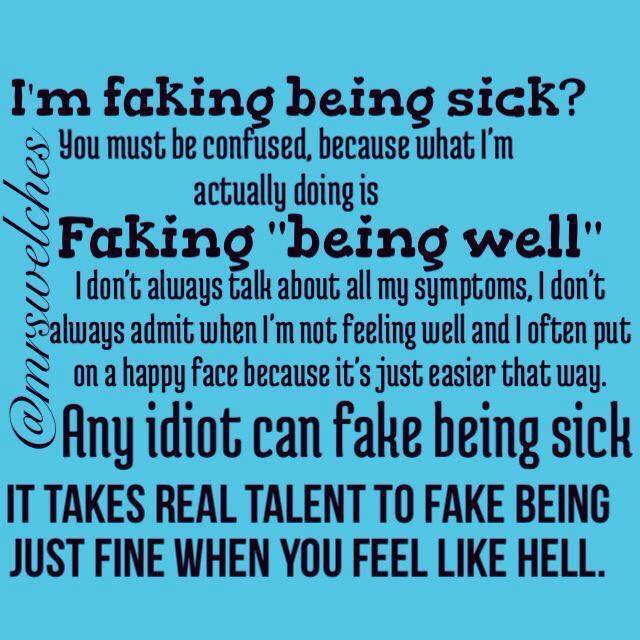The image is a square card with a blue background and black text, addressing the complexities of faking wellness despite feeling unwell. The text begins in large black letters with "I'm faking being sick?" and continues in smaller letters, "You must be confused because what I'm actually doing is," followed by large, bolded text, "faking being well." "Being well" is in quotation marks. The message goes on to explain, "I don't always talk about all my symptoms. I don't always admit when I'm not feeling well, and I often put on a happy face because it's just easier that way." It concludes in large, bolded text, "Any idiot can fake being sick. It takes real talent to fake being just fine when you feel like hell." The social media handle "@mrs.welch's" is noted on the card. The text varies in font size and boldness to emphasize different parts of the message.